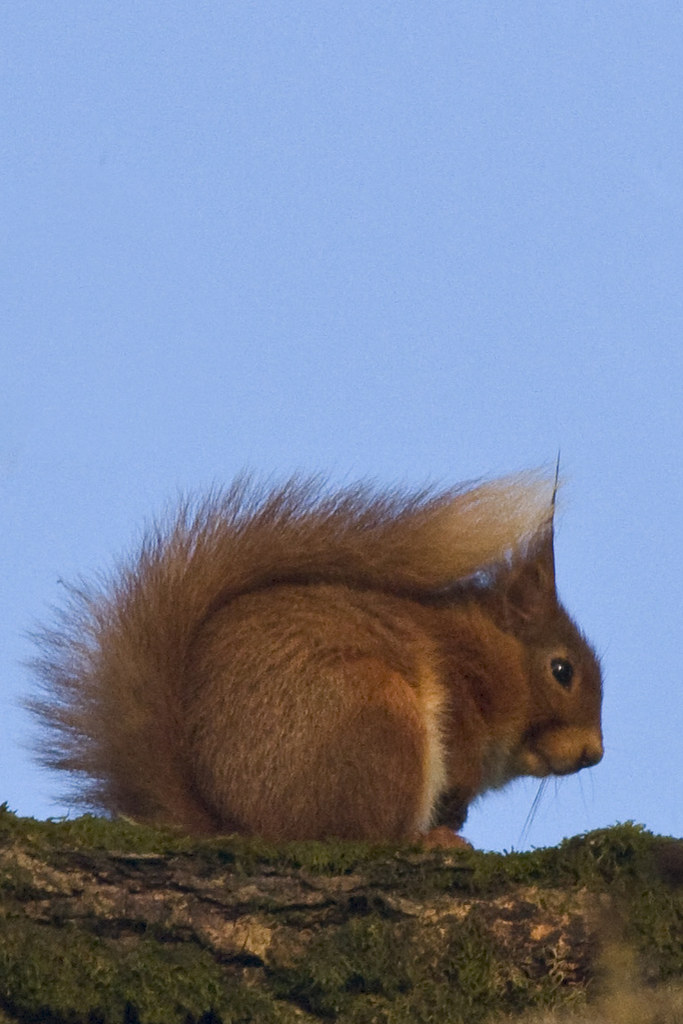This is a detailed and descriptive caption combining the elements from both voices:

This photo captures a cute, fuzzy brown squirrel perched on a mossy log. The squirrel is shown in profile, with its right side visible and its tail resting on its back. Its large eye and nose are noticeable as it stares to the right. The sky is clear and blue, providing a vibrant backdrop. The squirrel appears slightly unhappy, hunched over as if it's cold. The log or branch beneath it is covered in moss, adding to the natural setting of the photograph.